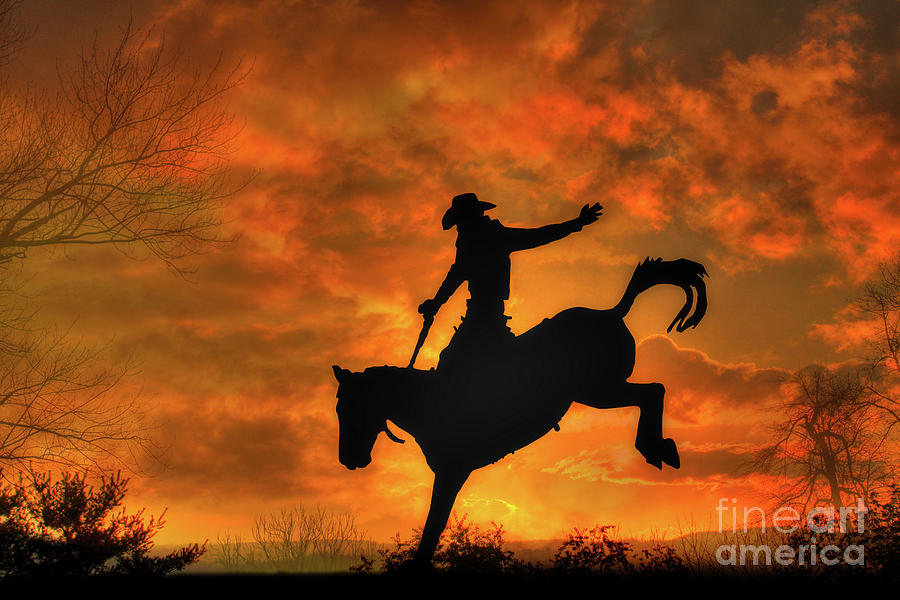In this striking digital illustration, the focal point is a dramatic silhouette of a cowboy on a bucking horse, reminiscent of a scene from a rodeo. The horse's back legs are kicked high in the air, with its front legs planted firmly on the ground, capturing a moment of intense action as the cowboy holds on with one hand, his other hand raised high, clutching the reins. Both horse and rider are rendered in stark black, creating a powerful contrast against the vivid, fiery background. The sky is awash in blazing hues of orange, red, and brown, with swirling clouds that enhance the sense of movement and drama. The sun appears to be setting, casting an intense light that almost seems to set the sky on fire. On either side of this dynamic scene, barren trees and bushes frame the composition, adding elements of depth and texture. In the bottom right corner, white text reads "Fine Art America," indicating the source of this evocative artwork.